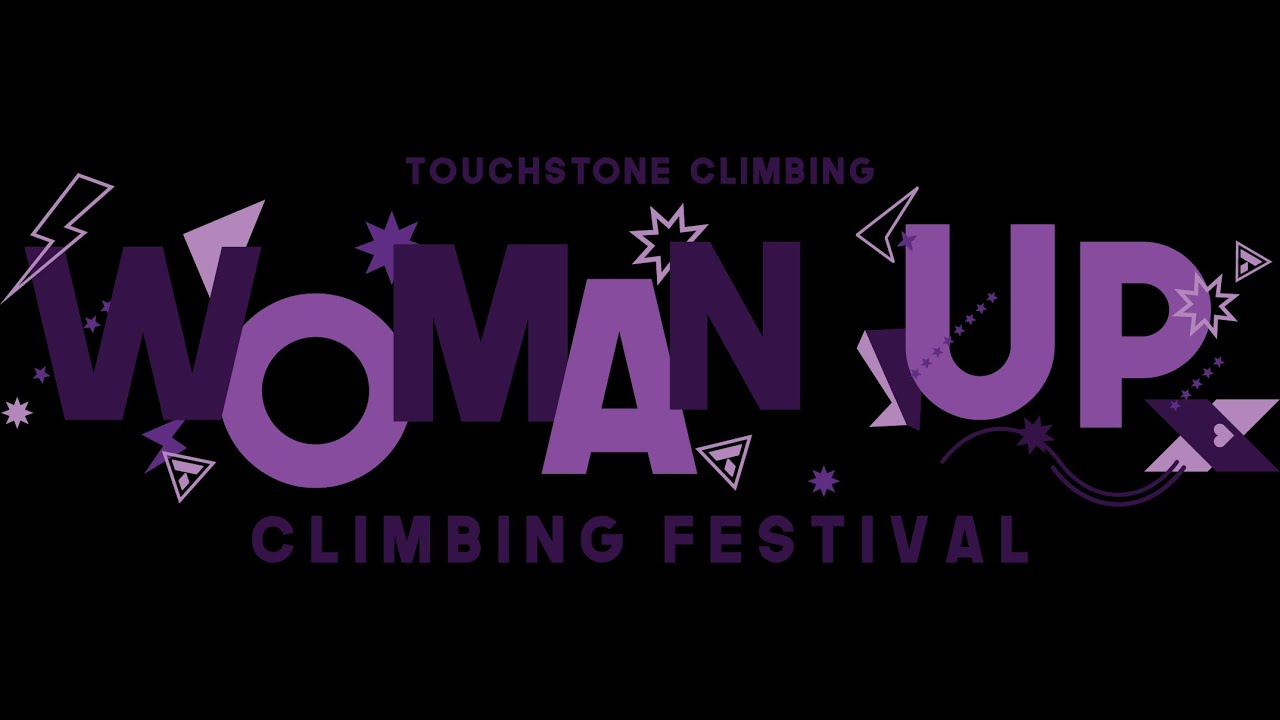The image is a rectangular graphic design, approximately five inches wide and three inches high, featuring a minimalist and geometric style with a black background. At the top center, in small purple print about an eighth of an inch high, are the words "Touchstone Climbing". Below that, the main title "Woman Up" is prominently displayed in large print with alternating light and dark purple letters: the W is dark purple, the O is light purple, the M and N are dark purple, and the A, U, and P are light purple. Surrounding the title are small illustrations of lightning bolts, stars, check marks, boomerangs, triangles, and a heart. Below the main title, in medium-sized dark purple print, the words "Climbing Festival" are displayed. Overall, the composition features a dynamic arrangement of text and symbols, contributing to the design's energetic and celebratory feel.